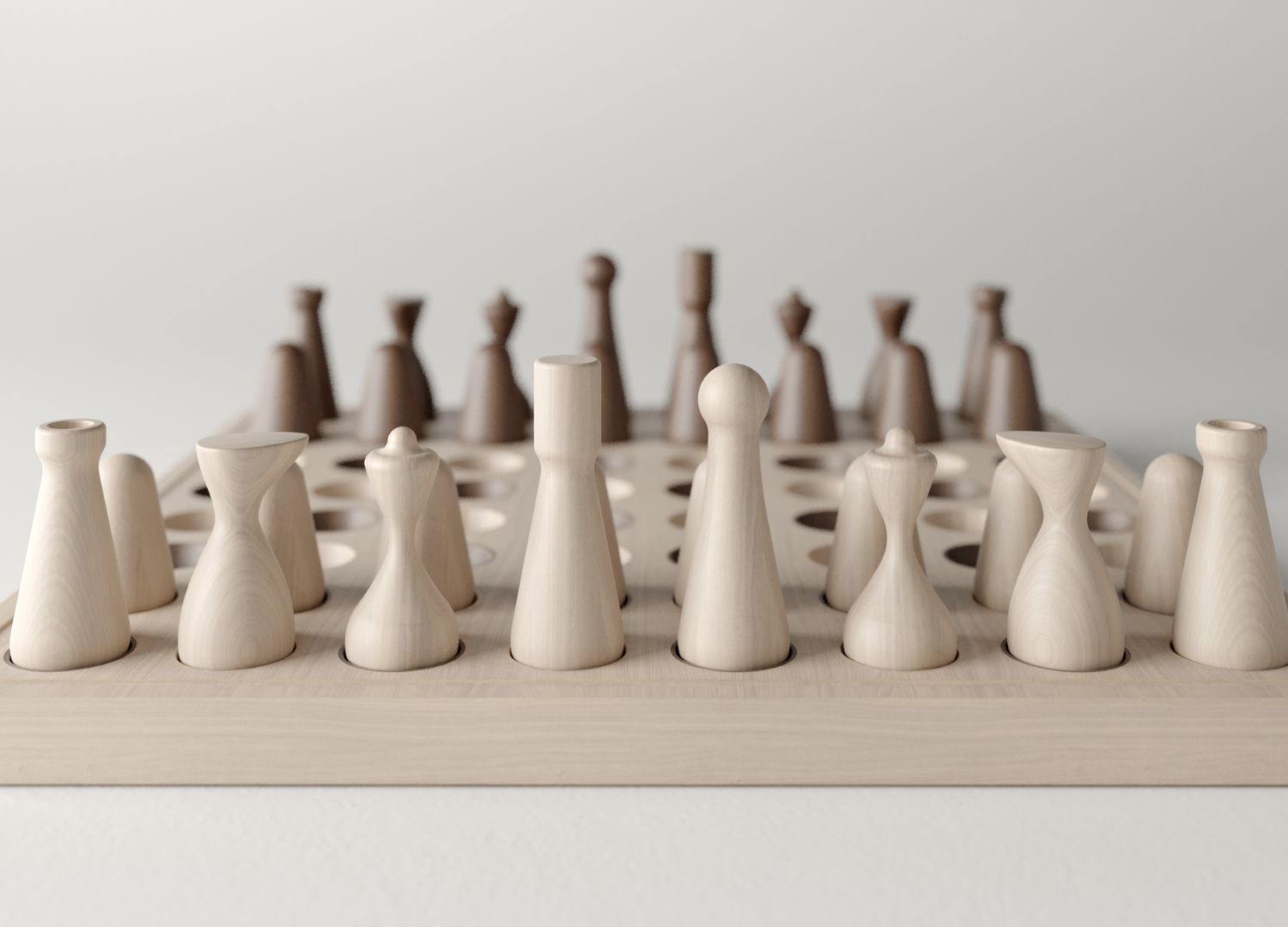This image showcases a finely crafted wooden chess set featuring a unique and modern design. The chess pieces, differentiated by their simplistic and smooth appearance, are divided into two groups: light beige pieces on one side and dark brown pieces on the other. Each piece is meticulously placed within hollowed-out grooves on a flat, light beige board, which adds to the set's contemporary aesthetic. The board itself is unobtrusive yet elegant, with small holes to accommodate the pieces, allowing for an organized and streamlined look. The background of the image is a soft gray, providing a subtle contrast that highlights the intricate details of the chess set. This daytime photograph captures the minimalist beauty and functional artistry of the game.